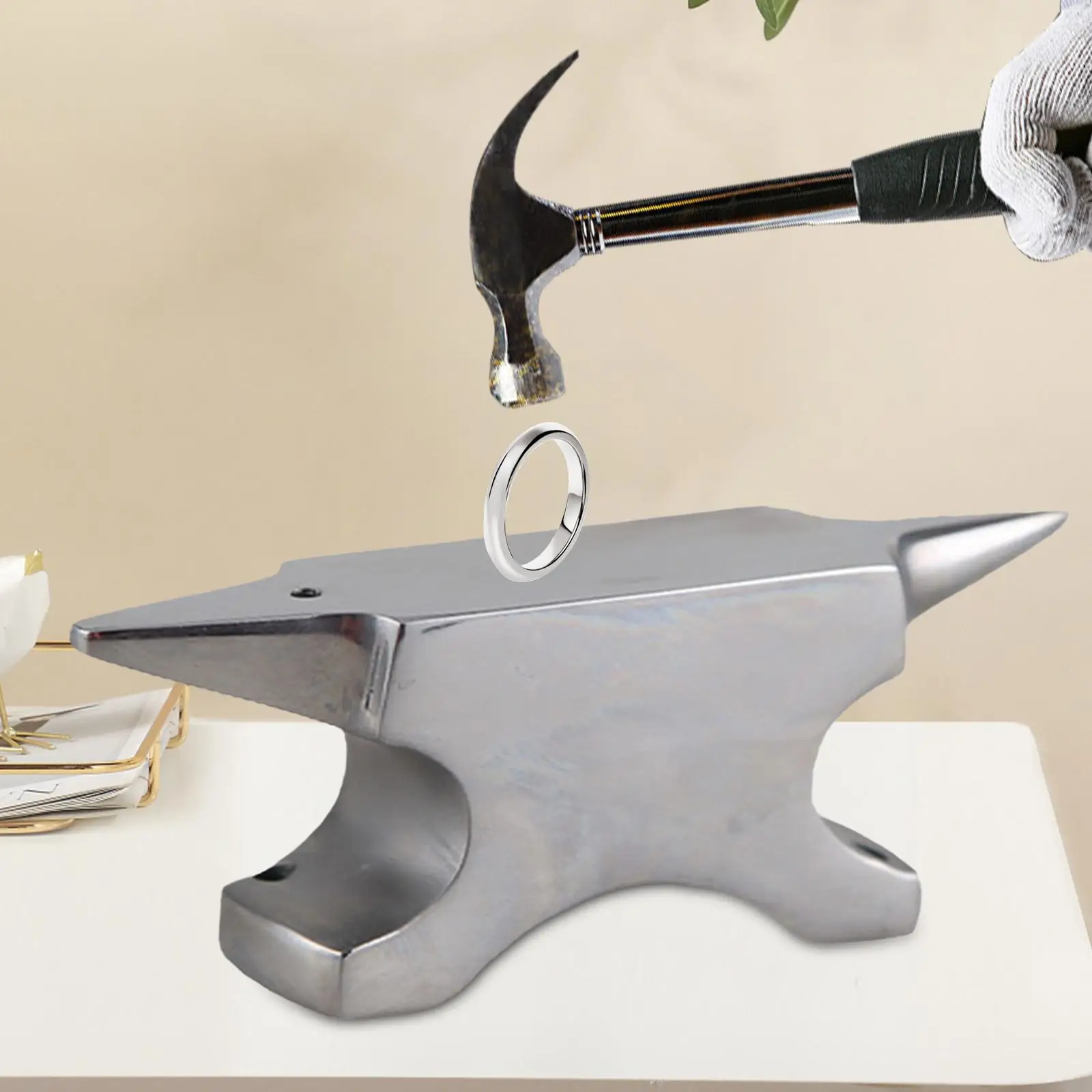The image is a digitally manipulated scene depicting a large, shiny silver anvil placed on a white table against an off-white wall background. A sizeable white wedding ring, larger than normal finger rings, is positioned upright on the anvil. A man wearing white garter gloves holds a black and silver hammer, poised mid-swing above the ring. The composition appears to have been edited, as the elements look artificially arranged and stylized. On the left side of the table, various envelopes or papers are scattered. The overall scene, including the anvil and the hammer, has a new and polished appearance.